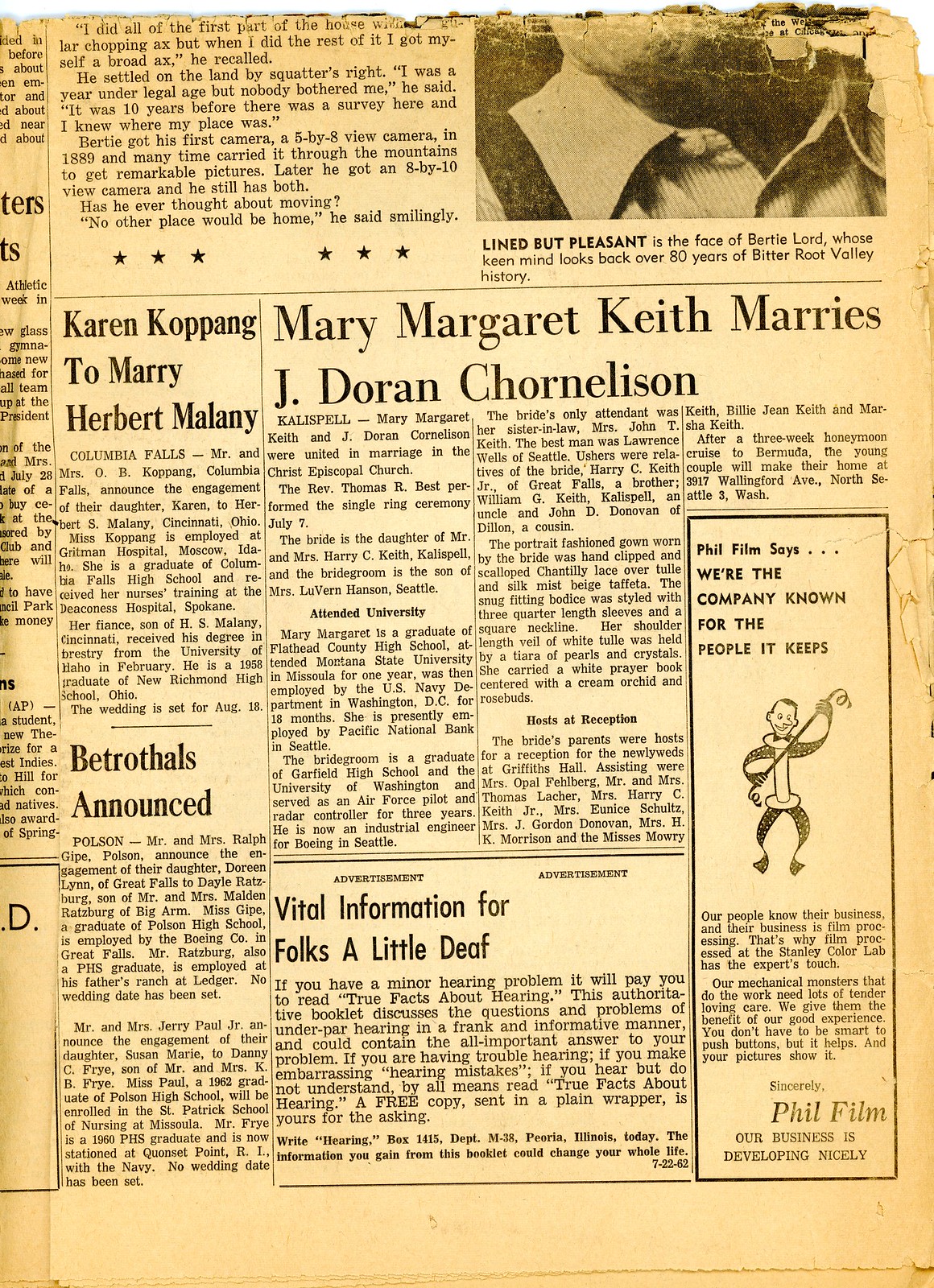In this image, we see an aged, yellowed section of a newspaper that appears to have once been white. The newspaper features a variety of stories and advertisements. On the top left, there is a story that is partially cut out, making it difficult to read. Moving towards the center left, there is an announcement detailing the upcoming marriage of Karen Copping to Herbert Malaney. Adjacent to this on the right, there is another wedding announcement involving Mary Margaret Keith and Jade Chornelson.

Beneath these announcements, several other features are visible. Below the first marriage announcement, there is a segment titled "Bit True Dolls Announced," though the rest of the text is unclear. Another story under the second marriage announcement is titled "Vital Information for Folks a Little Deaf."

On the far right side, there is an advertisement for a company named Phil Film. The ad contains a drawing of a man and includes the tagline, "We're the company known for the people it keeps." It is signed off with "Sincerely, Phil from Phil Film," and ends with the line, "Our business is developing nicely."